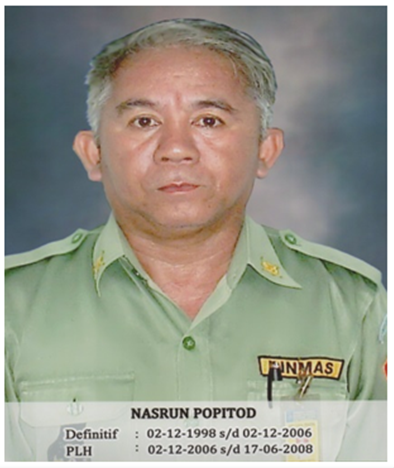The photograph depicts a gentleman named Nasrun Poppy Dodd, also referred to as Nasrin Popatad or Nazran Papatad, standing and facing forward in an official or military-like green outfit. His attire, which could suggest a naval or managerial role, features shoulder lapels, green buttons, and a yellow nameplate partly obscured by pens in his shirt pocket. This nameplate includes his name and possible service dates: 02-12-98 to 02-12-206 and 02-12-206 to 217-6-2008. The gentleman appears to have Filipino origin, with black eyes, fair skin, and gray hair. Yellow patches adorn his neck collar, and the background of the image is cloudy. The photo, conveying a straightforward and almost mugshot-like pose, hints at legal or definitive purposes.